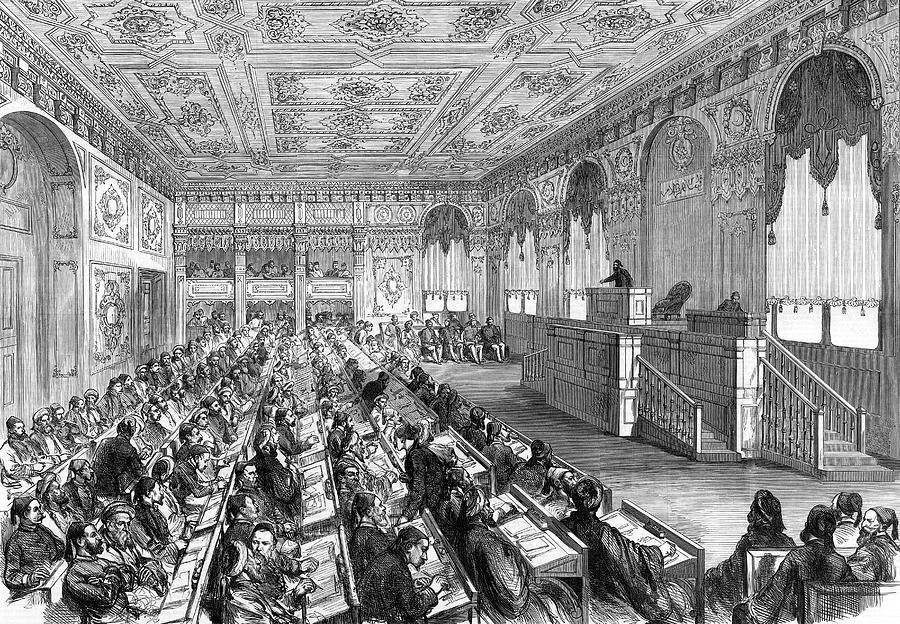This detailed black and white etching depicts a grand, rectangular room with a tall, ornate ceiling and intricately carved decorations. At the front of the room, a raised podium, accessible by stairways on either side, features a man dressed in black addressing a large assembly. The audience, comprising mostly older men, sit at rows of desks equipped with angled surfaces for writing, some actively taking notes while others listen attentively or engage in quiet conversation. The right wall is lined with tall windows adorned with elaborate curtains. In the background, an ornate back wall with a large door is visible, and above it, a balcony where additional spectators observe the scene. The setting exudes a Romanesque architectural influence and the atmosphere is reminiscent of a formal gathering, possibly a lecture, court session, or government meeting.